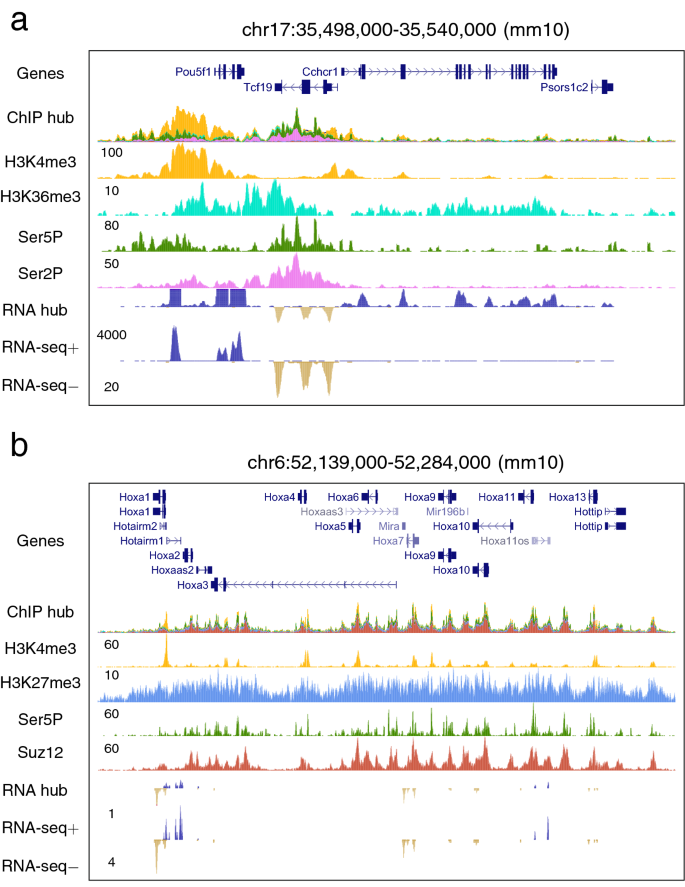The image depicts an intricate genetic breakdown presented against a solid white background, featuring two stacked rectangular charts labeled A (top) and B (bottom), each containing color-coded line graphs representing various genetic and protein data. Both charts have a plethora of text on the left side, listing "Genes", "CHiP Hub", "H3K4Me3", "H3K36Me3", "Ser5P", "Ser2P", "RNA Hub", "RNA-Seq Plus," and "RNA-Seq Minus". Above Chart A, additional details include "CHR17, 35,498,000-35,540,000, MM10". The area graphs within both charts vary in color, displaying peaks and valleys in shades of yellow, green, pink, purple, and blue, illustrating the presence and levels of specific proteins associated with genes. Chart B is notably more populated with entries under the genes section, suggesting a deeper or broader analysis. Despite the absence of further context, the detailed depiction implies a focus on genetic sequencing data and related protein activities.